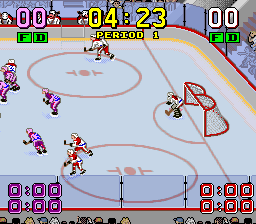The image is a low-resolution screenshot of an animated video game resembling old games from the 90s or 2000s, reminiscent of those on a Game Boy. It depicts an ice hockey rink, characterized by its simplistic, nostalgic graphics. The white ice surface has painted red goal areas and feature specific markings: two circles in the middle foreground each with the letter "T" inside. The rink is bordered by a barricade with a yellow line at the bottom where it meets the ice, and a red line at the top, topped with Perspex panels with visible joins for crowd protection.

In the scene are two competing teams, with players wearing distinct uniforms — four players in purple jerseys and four in orange and white jerseys, all holding black hockey sticks. The hockey nets have red poles and black hash lines. Above the rink, the scoreboard displays 00 in purple with the letters FD in black on a green background underneath and the time 04:23, indicating the first period. Another score display reads 00, also with FD in black letters on a green background below.

In the foreground, the heads of spectators are visible, adding to the immersive, albeit retro, gaming atmosphere.